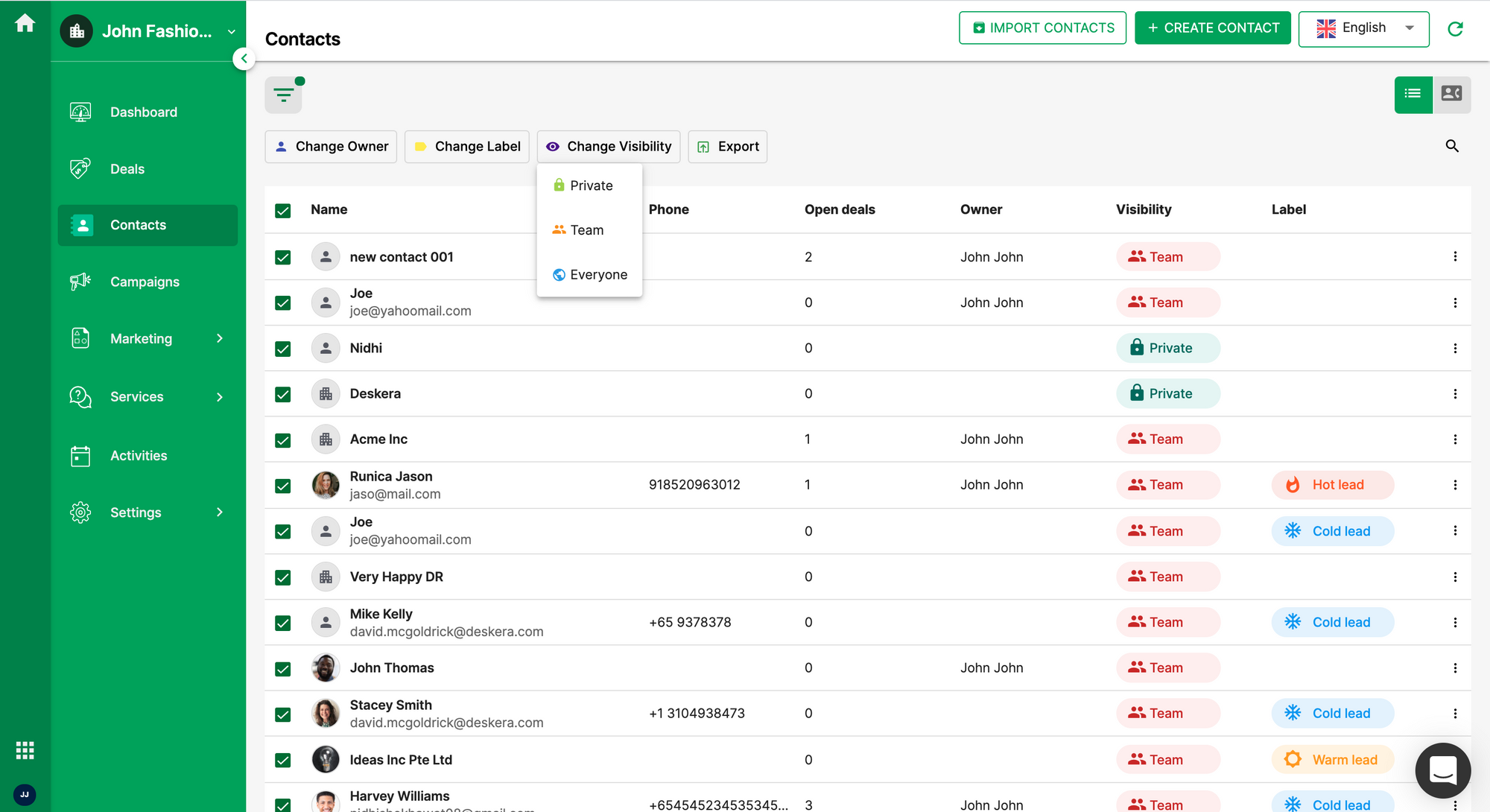The image is a detailed screenshot from a user interface of what appears to be a web-based application or CRM (Customer Relationship Management) software. The layout features a green theme, with a vertical navigation menu situated on the left side, spanning from the top to the bottom of the screen. This menu contains various options such as "Dashboard," "Deals," "Contacts," "Campaigns," "Marketing," "Services," "Activities," and "Settings," each accompanied by matching white icons. 

At the very top of this menu, there is an icon that seems to represent a home or apartment, next to which the text "John FASIO..." is displayed in white. The "Contacts" option is highlighted in a darker green box, indicating it is currently selected.

The main area of the screen is dominated by a large interactive table designed to manage contacts. At the top of this section, just below the menu, there are buttons and icons including "Import Contacts," "Create Contacts," a filter icon, a three-lines icon indicative of a more options menu, and a person icon. Another interactive button allows users to change owner, labels, and visibility settings. The visibility setting is currently open, showing choices such as "Private," "Team," and "Everyone."

Further below, the main table is organized like a spreadsheet, featuring columns for Name, Phone, Open Deals, Owner, Visibility, and Label. Some rows include profile pictures or default icons, and the visibility statuses are color-coded, with "Team" displayed in red and "Private" in green. Labels are also included, color-coded as hot leads, cold leads, and warm leads next to various contact names and details.